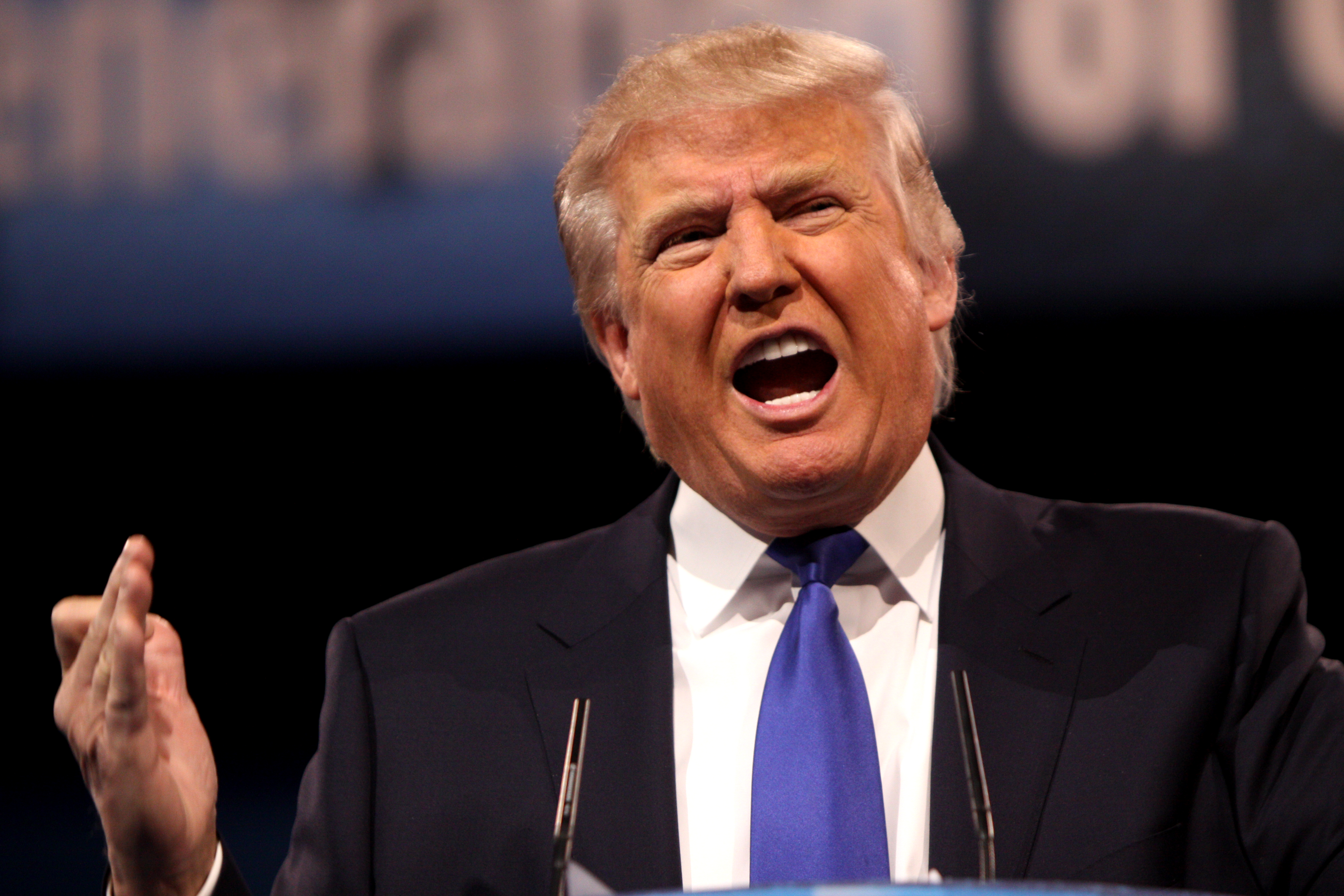This photograph captures Donald Trump mid-speech, standing at a podium equipped with two small black microphones jutting from the top. Dressed in a dark suit with a white dress shirt and a blue tie, Trump appears to be speaking forcefully, as indicated by his wide-open mouth and intense expression. His right hand is raised and gesturing, with the thumb and index finger almost touching while the other three fingers point outward. His eyes are slightly squinted, adding to the intensity of his expression. His hair, a distinctive orange-ish blonde, contrasts against the backdrop, which features a blurred blue-to-black gradient with indistinct white text that cannot be read. Although Trump faces forward, his gaze is directed slightly to his right, emphasizing his dynamic presence as he engages with his audience.